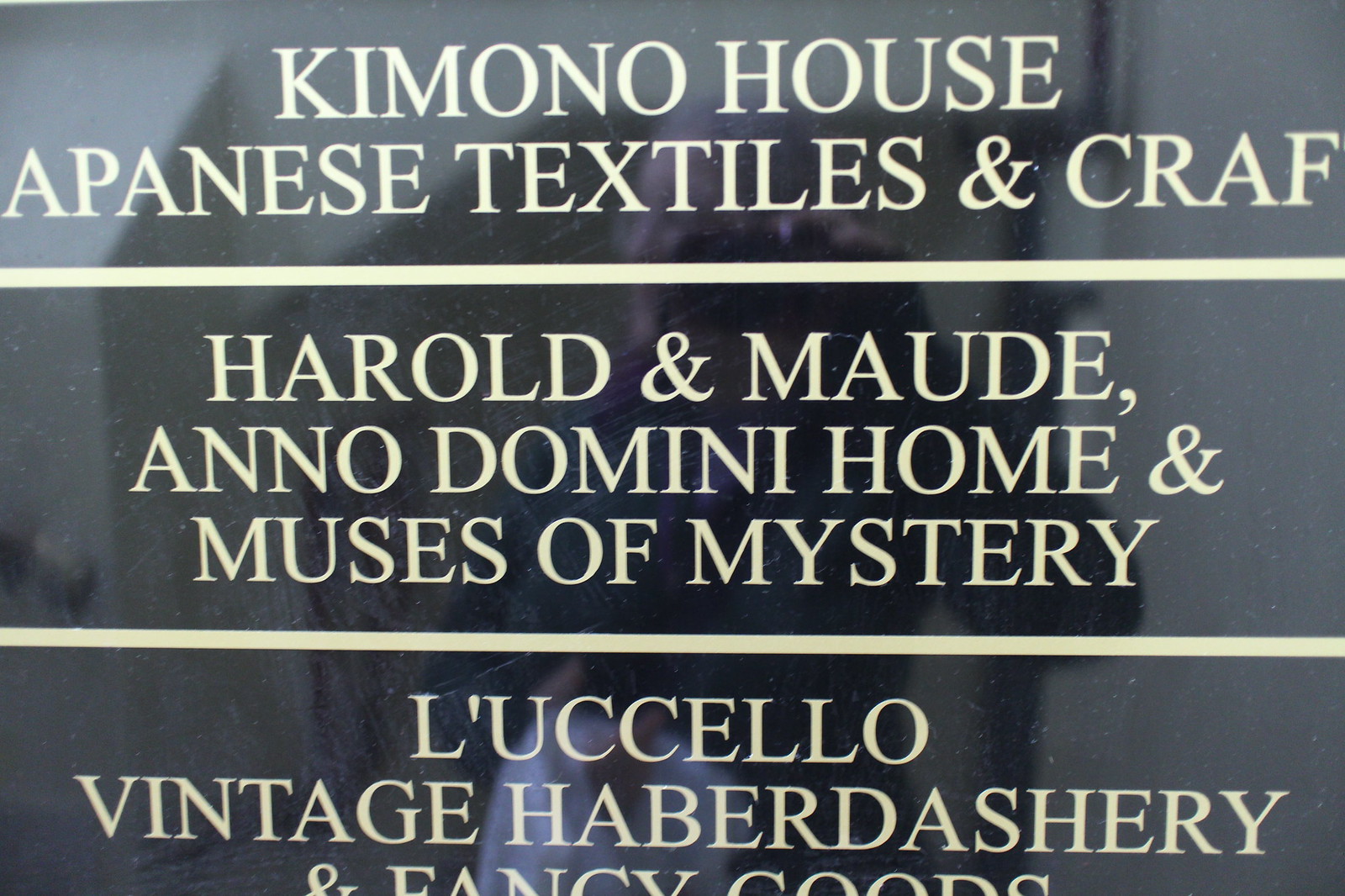The image captures a photograph of a glossy, black stone advertisement mounted on a wall, illuminated with a slight glare. The advertisement, primarily featuring uppercase letters in a cream yellow or light goldish color, is organized into three distinct rows, each separated by lines. At the top center, the sign reads "KIMONO HOUSE," followed by "JAPANESE TEXTILES AND CRAFT," though the beginning letters 'J' and 'T' are partially cropped. The middle row lists "HAROLD AND MAUDE," "ANNO DOMINI HOME," and "MUSES OF MYSTERY." The bottom row displays "LUCCIELLO VINTAGE," "HABERDASHERY," and "FANCY GOODS," with the latter partially cut off at the bottom edge of the photo. Centrally reflected in the polished surface of the sign is the silhouette of the person taking the picture. The upper left corner of the image shows a white wall with an indentation and its accompanying shadow.